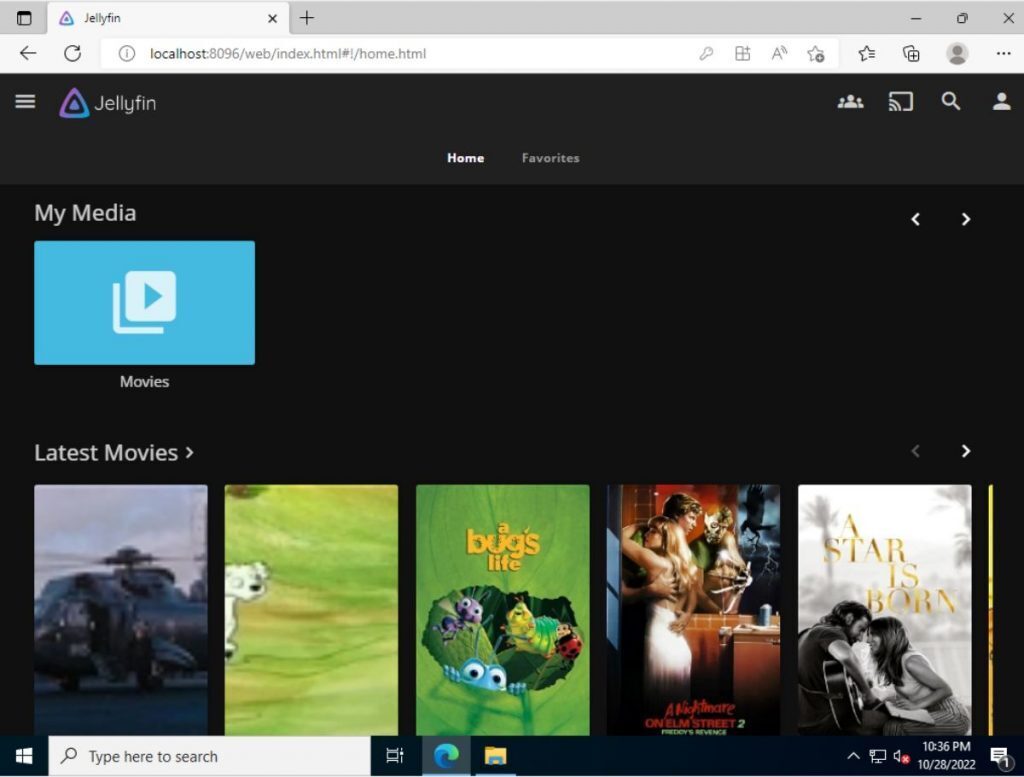Here is a polished and detailed caption for the image:

---

The image showcases a web browser page with the URL "localhost:8096/web/index.html" displayed in the address bar. The webpage loaded is the interface of Jellyfin, a media server application. Positioned on the top left corner, the Jellyfin logo features two overlapping triangles with a gradient transition from purple to blue. The background is predominantly black, with white text providing clear contrast.

Central to the interface are two prominent tabs labeled "Home" and "Favorite". In the top right corner, a set of icons is aligned horizontally: a group icon, a screencast icon, a search icon, and a profile icon.

On the left side of the page, there's a section titled "My Media", under which a blue folder labeled "Movies" is displayed, accented with a white play button. Below this section, a category titled "Latest Movies" showcases a selection of the most recent films in a horizontal row of five thumbnails. 

- The first movie, positioned at the bottom left, features an image of a black helicopter.
- The second movie thumbnail shows a white goat against a green background.
- The third thumbnail is for "A Bug's Life," illustrated by a partially eaten leaf surrounded by four colorful bugs: purple, blue, green, and black with red accents. The movie title is prominently displayed in yellow at the top of the thumbnail.
- The fourth movie shown is "A Nightmare on Elm Street 2." 
- The fifth and final movie in the row is titled "A Star is Born."

---

This caption provides a detailed and structured description of the elements present in the image.